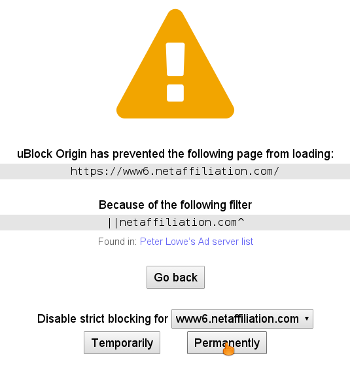In this detailed screenshot, the primary focus is a large gold triangle with a white exclamation mark at its center, signaling an alert or warning. Directly below this symbol, the message "uBlock Origin has prevented the following page from loading" is prominently displayed. Beneath this warning, a light gray banner includes the URL "https://www6.netaffiliation.com/".

Further down, the text "because of the following filter" appears, followed by another light gray banner containing "netaffiliation.com." Below this line, an additional note explains, "found in Peter Lowe's ad server list." Continuing down the image, another light gray banner with dark text offers a navigation option with the words "Go Back". At the bottom, there is an option highlighted within the tab labeled "Disable strict blocking for," followed by a space bar entry displaying "www6.netaffiliation.com." The overall design and messages reflect the actions and details pertaining to the browser's ad-blocking software, uBlock Origin.